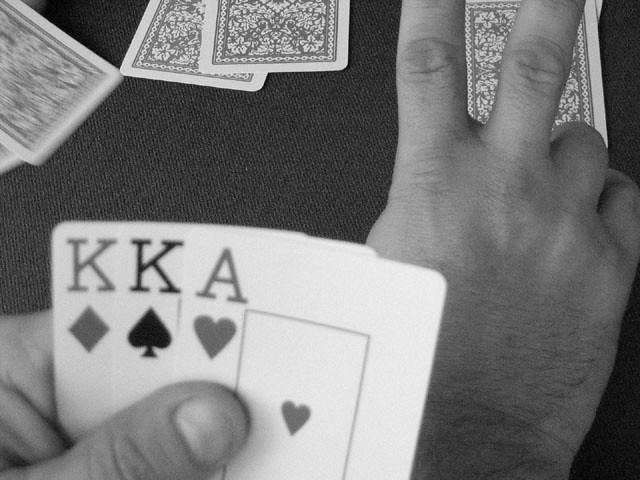A nostalgic black and white photograph captures the moment someone intensely focuses on their playing cards. The close-up shot highlights their left hand, positioned in the bottom left corner, delicately gripping three cards. The cards are an intriguing mix: the King of Clubs, the King of Spades, and the Ace of Hearts, with the Ace being fully visible. The gently curved thumb of the left hand is prominently seen, and it’s clear from the detailed texture that the hand is slightly calloused.

The right hand, situated just beneath the cards, forms a "peace" sign with the index and middle fingers extended, hinting possibly at a strategic or symbolic intention. Just beneath these fingers lies an additional card, face down on what seems to be a dark-colored tabletop, its color intensified by the monochromatic filter.

In the top left corner of the image, four more cards rest face-down, adorned with a heart or floral design on their backs and bordered elegantly. The setting evokes a sense of quiet tension and concentration, typical of a critical moment in a card game.